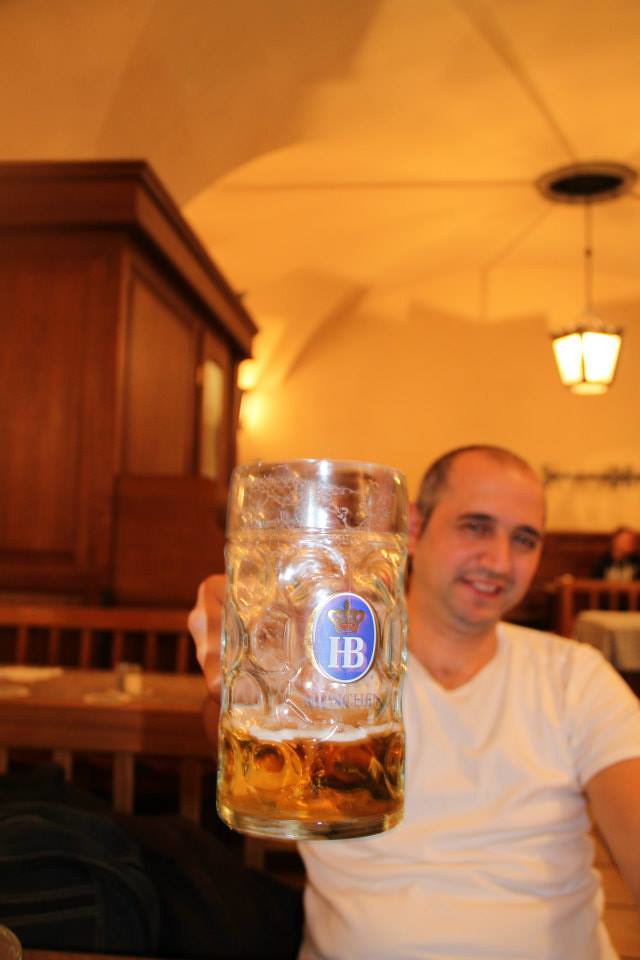In this detailed photograph, a smiling gentleman, likely in his mid-thirties, is prominently featured sitting in the Hofbräuhaus in Munich. He has a receding hairline and very close-cropped hair, and he is casually dressed in a white V-neck t-shirt. With his right arm extended in front of him, he holds up a glass beer mug, which appears to be mostly consumed, leaving about three inches of a dark golden amber beer. The mug displays a blue HB logo with a golden crown prominently on its front. Behind him, the backdrop includes a white ceiling with a single chandelier hanging from a black circular fixture, emitting a warm glow. Wooden furniture, including tables and chairs, populates the scene, but they are largely unoccupied save for one person sitting at a distant table behind the gentleman’s left shoulder. The setting conveys the cozy and sparse ambiance of the renowned beer hall.